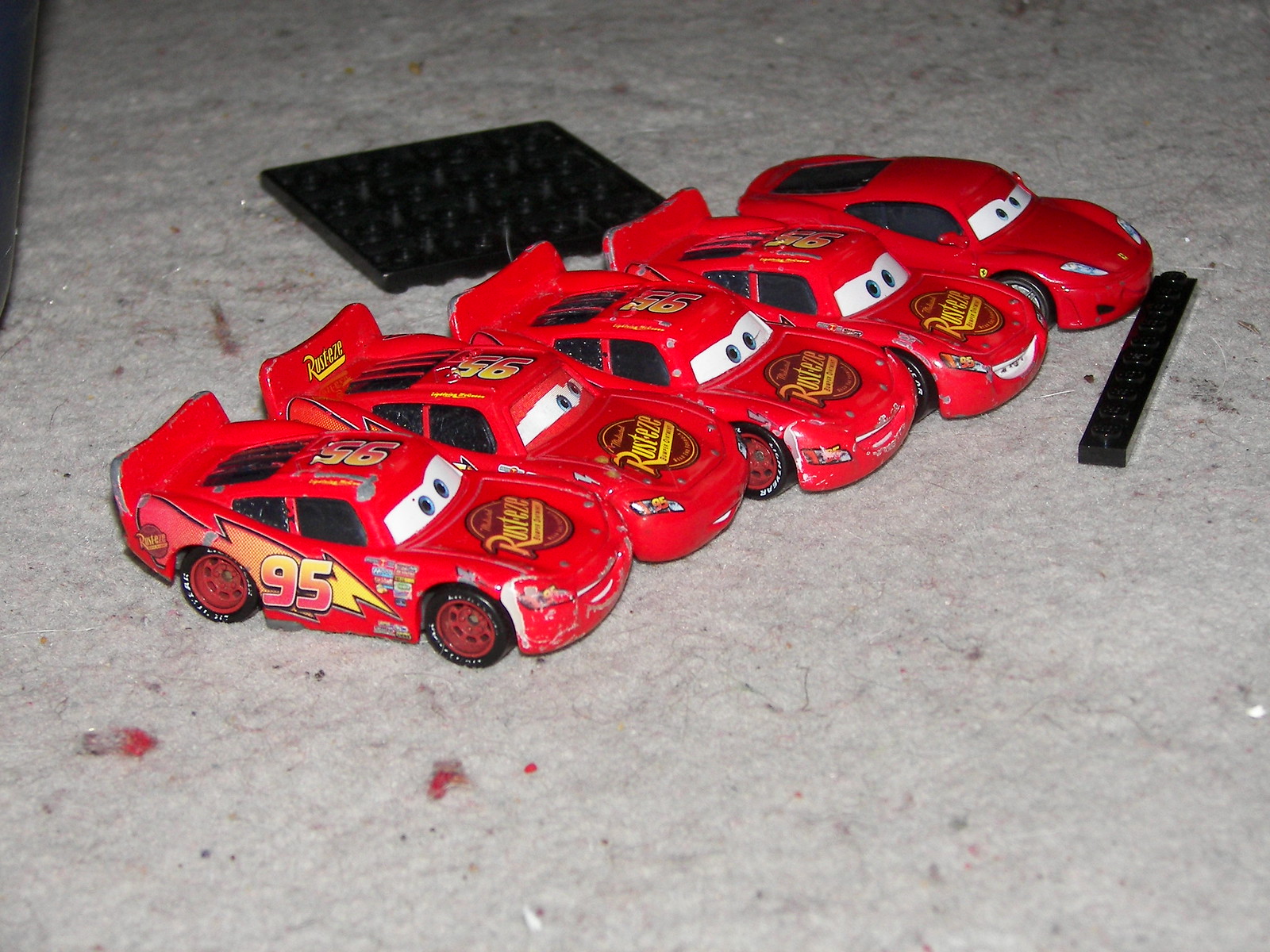This is a detailed photograph of five metal toy cars, each closely resembling the iconic character Lightning McQueen from the Disney Pixar movie "Cars." The cars are aligned diagonally from the lower left to the upper right on a gray surface, possibly a rug. 

All the cars are uniformly red sports cars with the number 95 in yellow on their sides overlaying a lightning bolt. Four out of the five cars also feature the same number on their roofs. These toy cars are detailed with cartoon eyes painted on a white stripe across the windshields, imitating the character's expressive eyes from the movie. The addition of black tires with red hubcaps and large spoilers at the back enriches their resemblance to the movie character. The frontal car also has "Rust-Eze" written on its spoiler and hoods.

The fifth car, however, stands out with some differences. Unlike the others, it lacks the number 95 on its roof and appears to be a plain red model with no additional markings or expressions beyond the eyes on the windshield.

The photograph includes a few peripheral details: a square black object behind the cars and a long rectangular black object in front, enhancing the scene's depth. The background seems to be decorated with tiny red spots, adding to the overall playful aesthetic of the image.